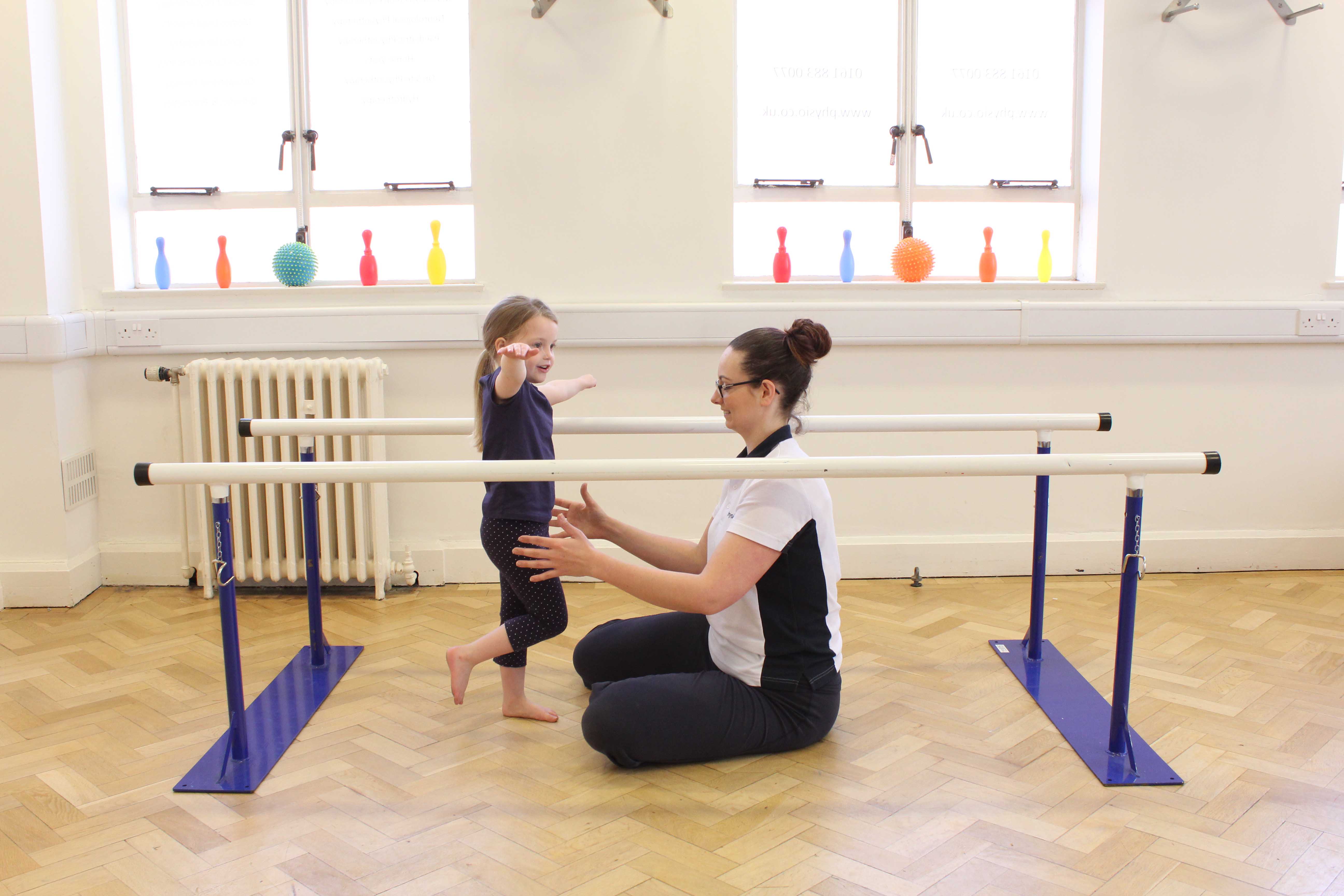In a brightly lit rehabilitation room with white walls and angled wooden panel flooring, a heartfelt scene unfolds. The room, equipped with therapy bars and adorned with lively knickknacks on the windowsills—including colorful plastic bowling pins and pumpkins—sets the stage for a touching moment of healing and support. A young girl with light brown hair pulled back into a ponytail proudly balances on her left foot, her right foot raised, and arms extended for balance. She is dressed in navy capri leggings and a matching t-shirt, flashing a joyous smile at the woman in front of her. 

The woman, a caregiver with brown hair neatly tied in a bun, sits on her legs and extends her arms, ready to catch the girl if she falters. She wears glasses and is dressed in a white and black short-sleeved shirt with black slacks. The therapy bars, white with black rounded tips, are supported by blue steel panels and stand as silent witnesses to this triumphant moment. In the background, two windows let in soft white light, further illuminating the room. The windowsills are lined with colorful, toy-like objects: plastic bowling pins in hues of blue, red, pink, yellow, and green, and similarly colorful balls, adding a whimsical touch to the clinical setting. This image captures a beautiful and hopeful moment within a therapeutic environment designed to assist children in regaining their mobility.